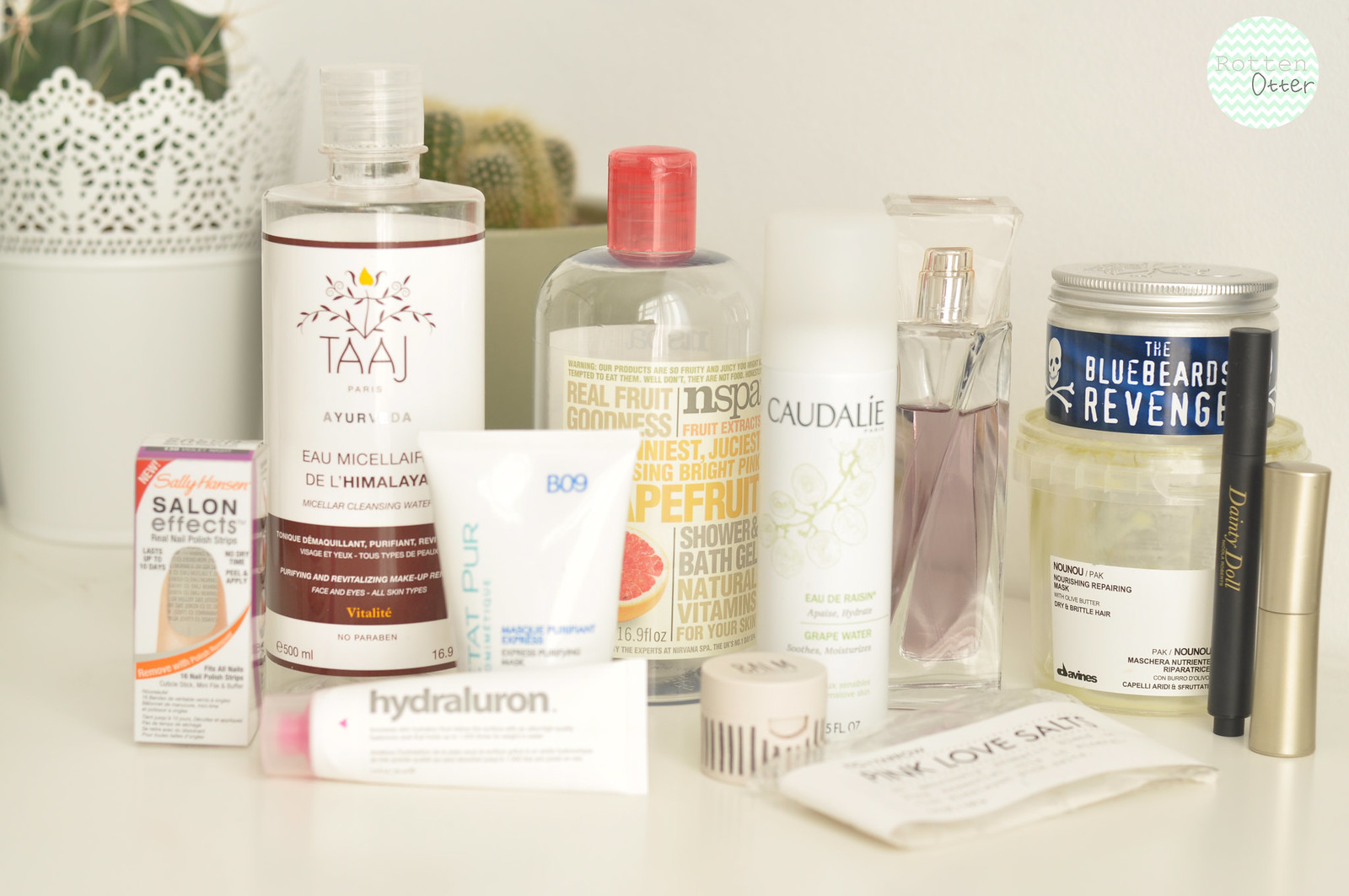This image appears to be an advertisement for various beauty supplies set against a clean, white background. At the back of the image, there are two white pots containing plants: a larger cactus on the left and a cluster of four smaller cacti slightly to the right of it.

In the foreground, there is an empty white box labeled "Salon Effects," suggesting it might be meant to hold other products featured in the image. In front of this box lies a tube of Hydraluron, likely meant to be stored in the box. Directly behind this, there is another white tube resembling a lotion container.

To the left, a large plastic bottle with a white label bordered in maroon at the top and bottom is prominently displayed. The label features the logo "Taj" and additional text that is hard to read.

On the right side, there is a clear bottle with an image of a grapefruit on it, adorned with a red lid and yellow text. Next to this, a tube labeled "Caudalie" sits in front of a small, circular MK-branded object.

Further to the right, a pink wrapper labeled "Love Salts" is positioned next to a clear glass bottle with a sprayer and pinkish-purple liquid inside. Behind this bottle, there is a jar with a blue label featuring a skull and crossbones, and the text "The Bluebeard's Revenge." Below this jar, another larger jar is partially visible, although its label is not entirely readable.

Finally, a black tube that appears to be eyeliner, although its text is unclear, sits next to a small silver lipstick, completing the array of beauty products displayed.